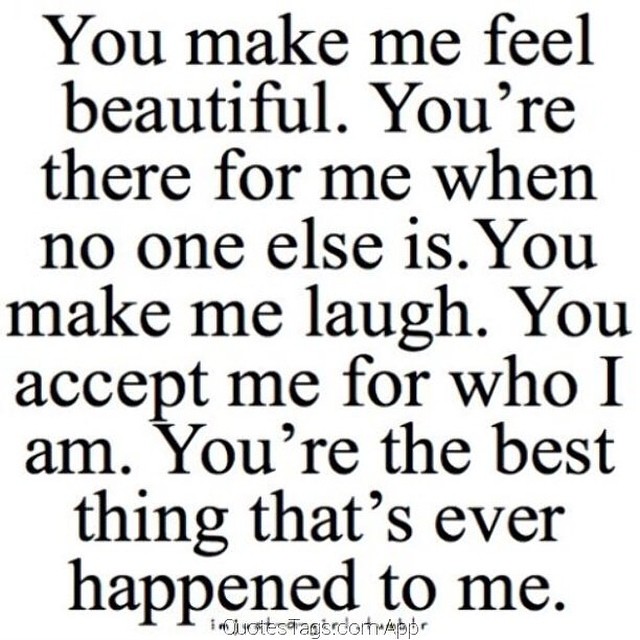This square-shaped image features a heartfelt quotation in centered, black Times New Roman font against a completely white background. The quote spans nine lines and reads: "You make me feel beautiful. You're there for me when no one else is. You make me laugh. You accept me for who I am. You're the best thing that's ever happened to me." At the very bottom center, there is a watermark in transparent blackish-gray font that reads "QuotesTags.com app." The overall design is simple yet impactful, emphasizing love and appreciation with straightforward, bold text.